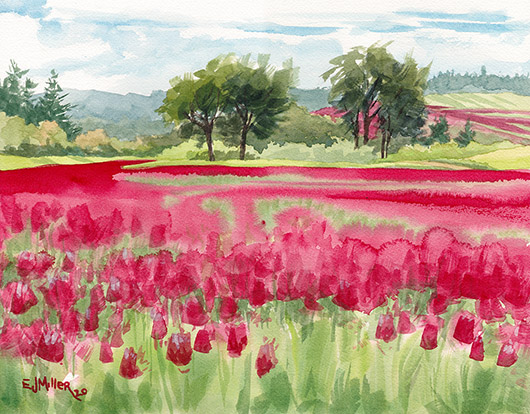This is a vibrant, colorful watercolor painting depicting a scenic flower field. In the foreground, red tulip and rose-like flowers blend with green stems and grass, creating a vividly detailed display. As you move further back in the image, the flowers merge into a blur of red swirls and splotches, forming a sweeping pattern across the field. The midsection of the painting showcases the same red hues in a more abstract manner, leading to the background, which features a line of tall trees. Some trees have brown trunks and green foliage, while others are entirely green, resembling pine trees. Above, the sky is predominantly cloud-covered with hints of light blue peeking through. The serene landscape is punctuated by a signature in the lower left-hand corner that reads "E.J. Miller, 20," indicating the artist's identification. This painting's dreamy and somewhat abstract style captures the essence of a bright, lively outdoor scene.